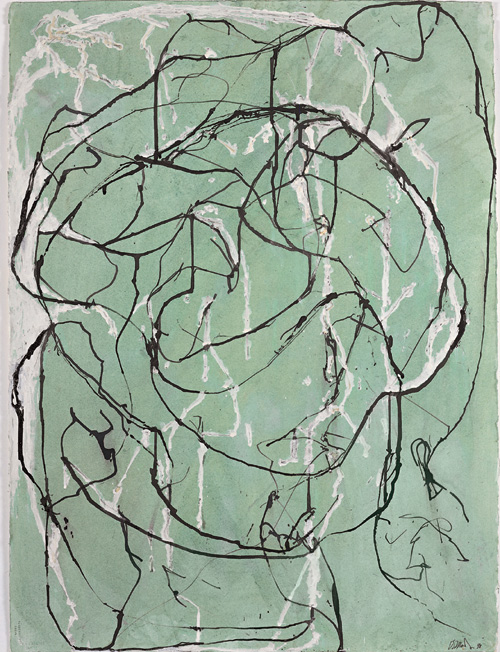This abstract painting features a variegated background in shades of medium and light olive green, creating a layered effect reminiscent of weathered surfaces. The backdrop is punctuated with wide, crackling brush strokes of white and gray, akin to marble veins, adding depth and texture. Across this complex background, thin, irregular black lines crisscross haphazardly, evoking images of tangled barbed wire or erratic drips of paint. These black lines intermingle with thicker, grayish-white strokes, further enhancing the painting’s chaotic yet organic feel. In the lower right corner, a barely legible artist’s signature can be found, marking the piece with a final touch of mystery.